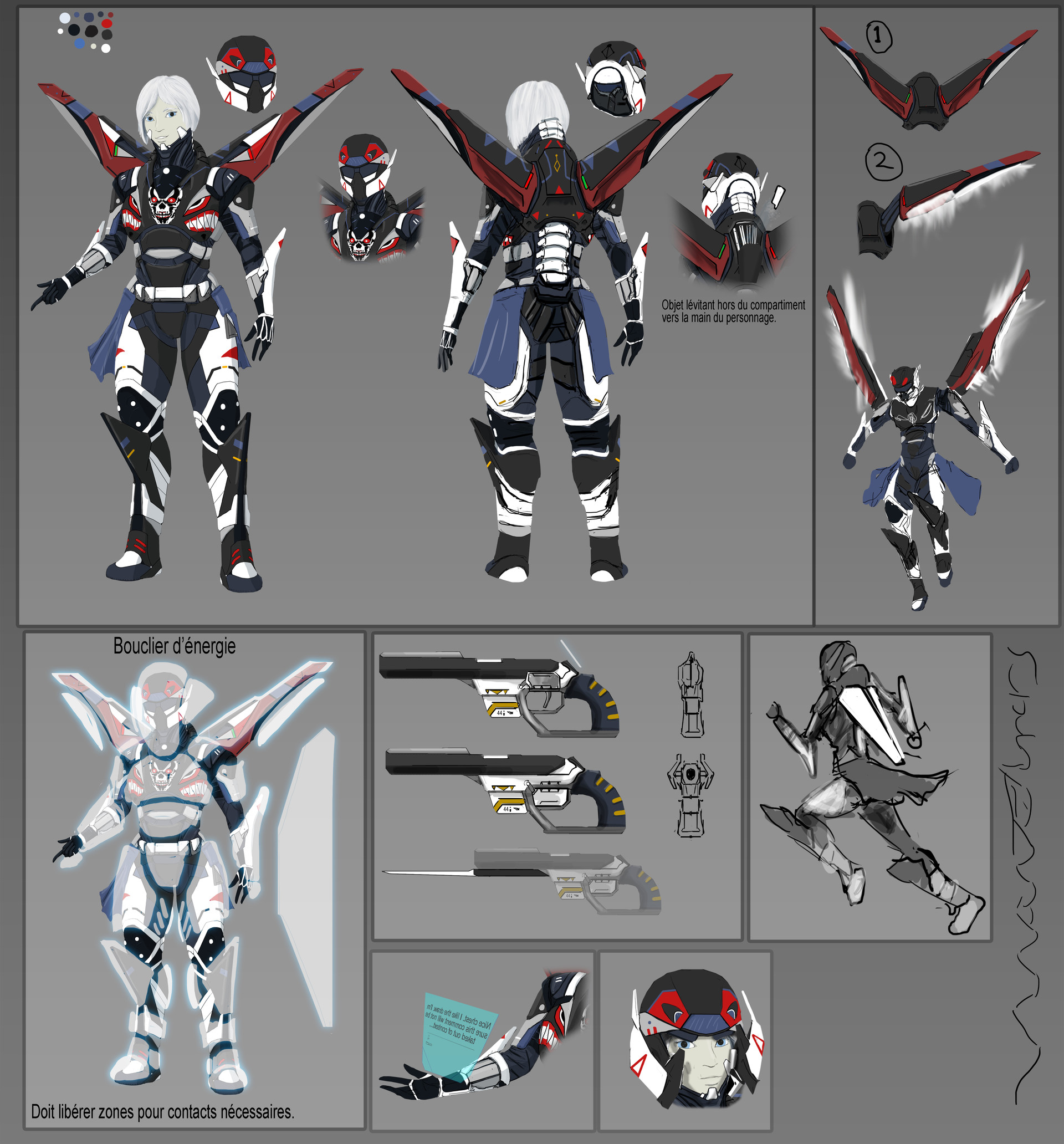This detailed concept art showcases a female character adorned in a sleek black and blue armor, designed to resemble a cutting-edge spacesuit. Her long white hair cascades just below her ears, complementing her sharp, space-age aesthetic. The full-body armor covers her from neck to feet and includes a helmet that can obscure her face. Notably, the shoulders of her armor expand outwards to mimic wings, adding a distinct dynamic to her silhouette.

Accentuating her impressive form, the character boasts vibrant red wings, intricately detailed on the right side of the image. Additionally, the bottom section of the artwork elaborates on her futuristic equipment: an energy shield, a sophisticated gun with a black muzzle, yellow accents, silver trigger, and handle, and a holographic projection device that extends from her wrist to supply vital information.

Presented against a dark gray grid background, the image features numbered annotations and text in an unidentified language, meticulously dividing each detailed component into individual squares. The vibrant color palette of reds, blues, whites, and blacks echoes a strong influence from Japanese animation, evoking a striking balance between traditional artistry and modern sci-fi elements.